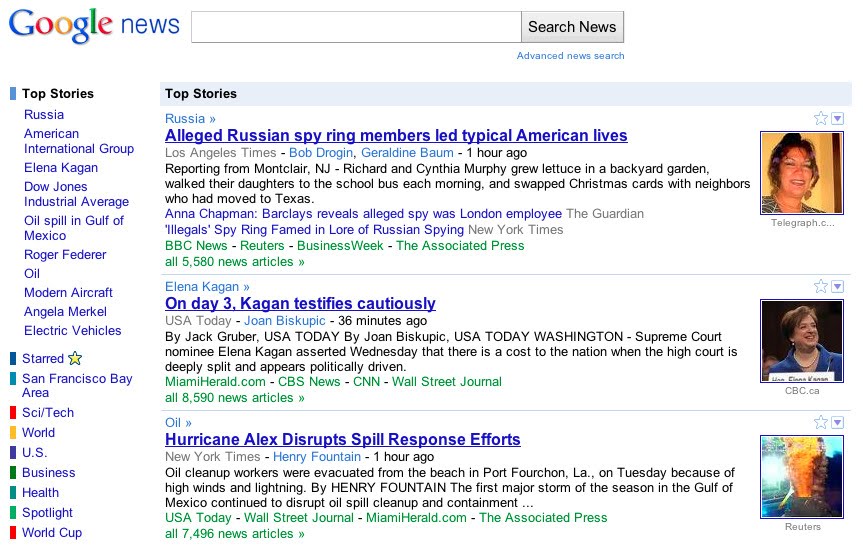This is a detailed description of a Google News search results page. In the upper left corner, the header displays "Google News." Centered at the top is an empty search box with the prompt "Search News" on its right side. Along the left-hand column, there is a list of sections arranged vertically, starting with "Top Stories," followed by individual topics such as "Russia," "American International Group," and "Elena Kagan." The sequence continues with "Dow Jones Industrial Average," "Oil Spill in Gulf of Mexico," "Roger Federer," "Oil," "Modern Aircraft," "Angela Merkel," and "Electric Vehicles." Further down, the list includes the word "Starred" accompanied by an image of a star, followed by "San Francisco Bay Area," "SciTech," "World," "U.S.," "Business," "Health," "Spotlight," and "World Cup."

On the main content area to the right, the section begins with "Top Stories." Below this heading, the first article title reads, "Russia." The accompanying headline states, "Alleged Russian spy ring members led typical American lives." The article is reported from Montclair, New Jersey, detailing that Richard and Cynthia Murphy grew lettuce in their backyard garden, walked their daughters to the school bus each morning, and exchanged Christmas cards with neighbors who had relocated to Texas. Adjacent to this article, on the right, is a square photograph of a woman with brown hair.

Following that, another headline appears titled "Elena Kagan." The subheading for this article says, "On day three, Kagan testifies cautiously." It emphasizes that Supreme Court nominee Elena Kagan remarked on Wednesday that the nation faces a cost when the high court is profoundly split and appears politically motivated. To the right of this article is a square photograph of a woman dressed in a blue outfit.

The final article headline reads, "Hurricane Alex disrupts spill response efforts." Next to this headline, on the right side, is a square image depicting a fire.